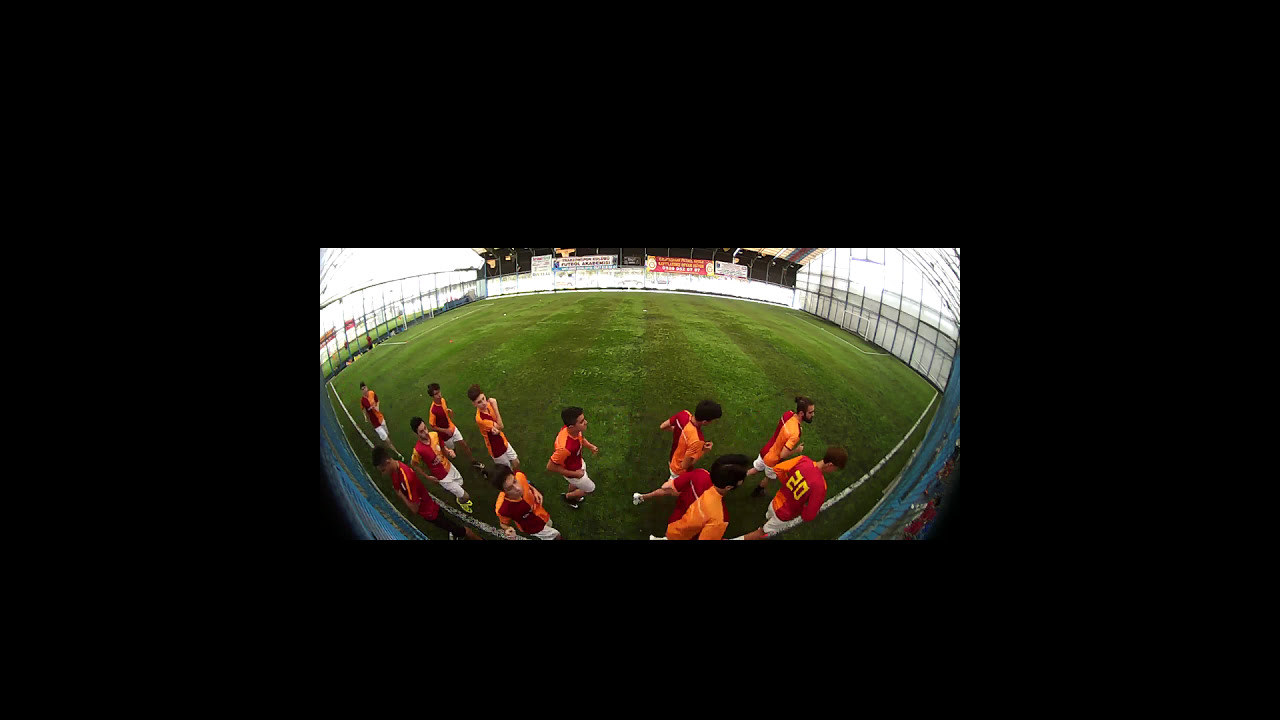The image depicts a panoramic view of a soccer field with light and dark gray grass stripes. In the foreground, a soccer team of eleven young men is jogging in pairs from left to right, wearing red and orange striped jerseys with white shorts. They are positioned on a curved, semi-circular path on the green pitch. The stadium walls encircle them, with spectator seating areas further up. A coach or manager stands on the side, observing. The scene is bright, with white light and black lines adding contrast. In the background, advertising billboards and goal nets are visible, along with some antler-like structures on the stadium's far wall. The overall effect is enhanced by a fishbowl lens, giving a raised and slightly distorted perspective.